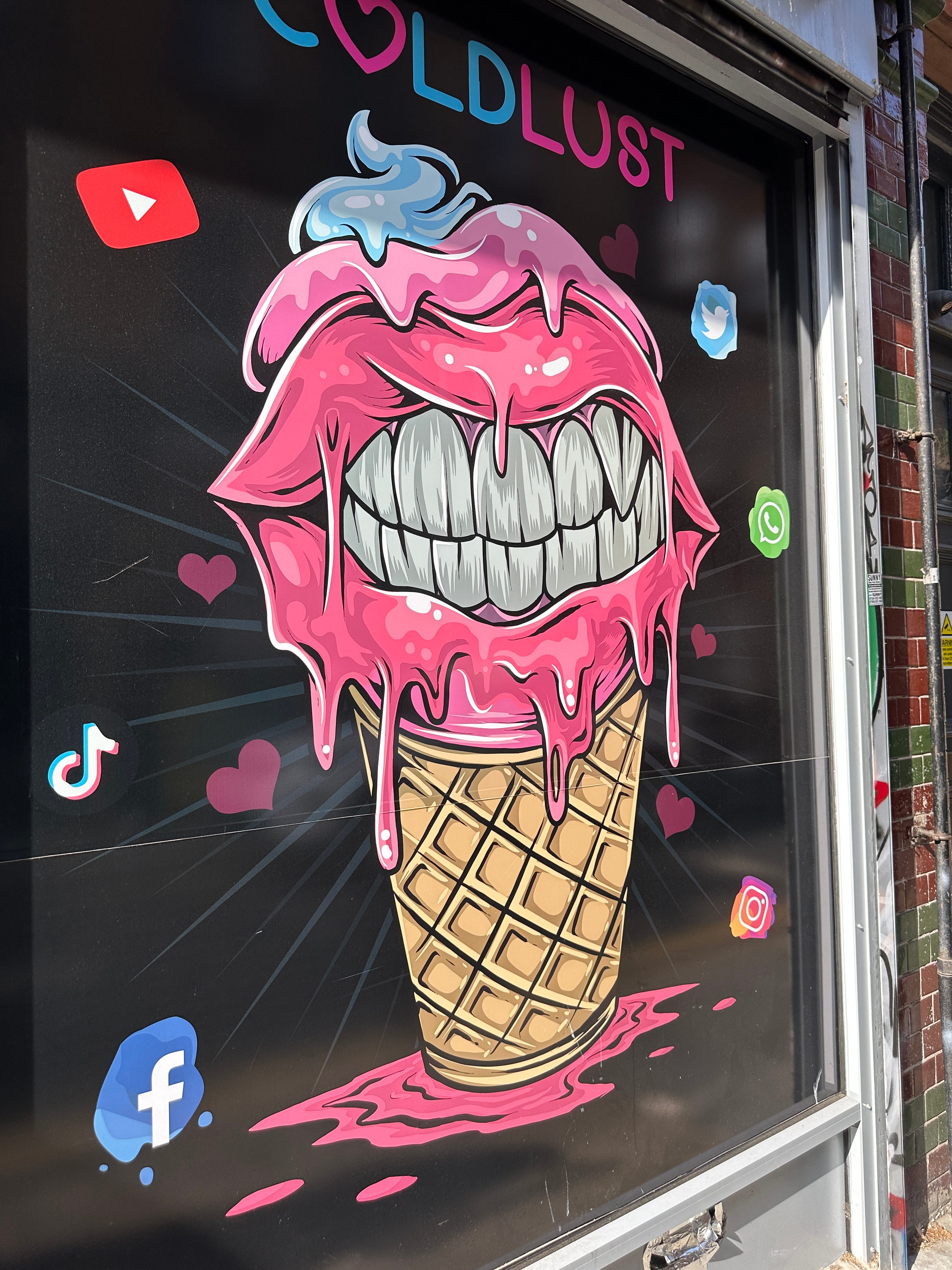This is a detailed photo of the front window of a storefront, likely an ice cream shop, decorated with a vibrant and cartoonish painting. The artwork features an ice cream cone with a brown checkered base and three scoops of ice cream: the bottom scoop resembles pink lips, smiling to reveal white teeth with a prominent upper left fang. The second scoop is a lighter pink, and the top scoop is a pastel blue. The ice cream is dripping and puddling around the bottom of the cone, giving it a dynamic appearance.

Above the cone, the words "Cold Lust" are written in a funky, handwritten, all-capital style. The letters are in blue and pink, with the 'O' replaced by a pink heart. Surrounding the artwork are various social media logos, including those of YouTube, TikTok, Facebook, Twitter, Instagram, WhatsApp, and more, creating a modern, connected feel. 

The image is set against a solid black background, enhancing the vivid colors, and to the right, there is a reddish-brown and gray brick wall, accented by metal tracks for a rolling gate that is open. The scene is lively with an eclectic mix of colors including black, white, gray, red, purple, pink, and yellow, making it a striking piece of window art.